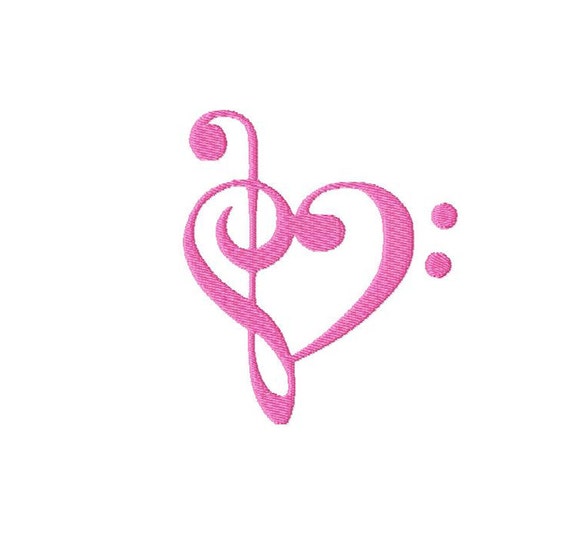The image features a detailed depiction of a pink, embroidered, musical symbol on a white background. Central to the design is a loopy, S-like figure that starts with a circle at the bottom, curves up and around, and then loops back in a complex, curving path. This central figure resembles a clef or a similar musical notation. The texture of the symbol is stitch-like, giving it a cloth or embroidered appearance. On the right-hand side of the symbol, there are two smaller, circular dots aligned vertically. The pink stitching stands out brightly against the clean, white background, emphasizing the intricacy and texture of the embroidered musical symbols.